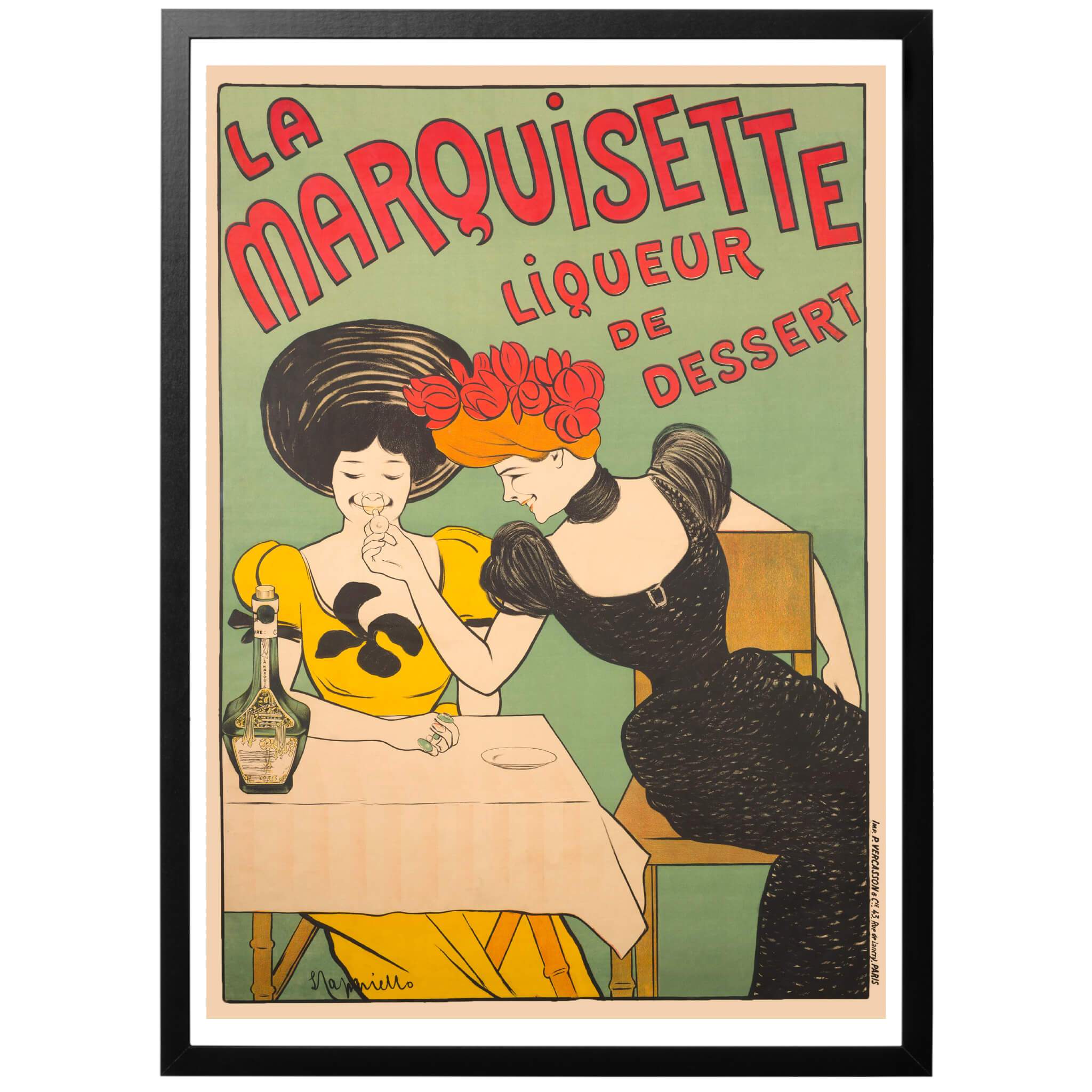The image is a vintage-style poster with a black frame, followed by a white inner border, and then a wood-textured rectangle encasing the main artwork. The central poster features a green background with the title "La Marquisette Liqueur de Dessert" written prominently in red at the top. The artwork depicts two animated women in Victorian attire. The woman on the left, seated at a table covered with a tablecloth, is wearing a yellow dress with a black ribbon and a black hat over her black hair. She has an intricate black decoration on her dress. The other woman, in a black gown with a scoop neck, orange hair adorned with red flowers, and a red hat, is leaning over from a chair next to the table and appears to be offering a tiny wine glass to the woman in yellow. A fancy green bottle, presumed to be gin, is placed on the table. The edges of the central image are framed by a pinkish border. The painter's name "Nepper Yellow" appears in the bottom left corner, while a vertical footnote "Yen Pi" is inscribed at the bottom right center.